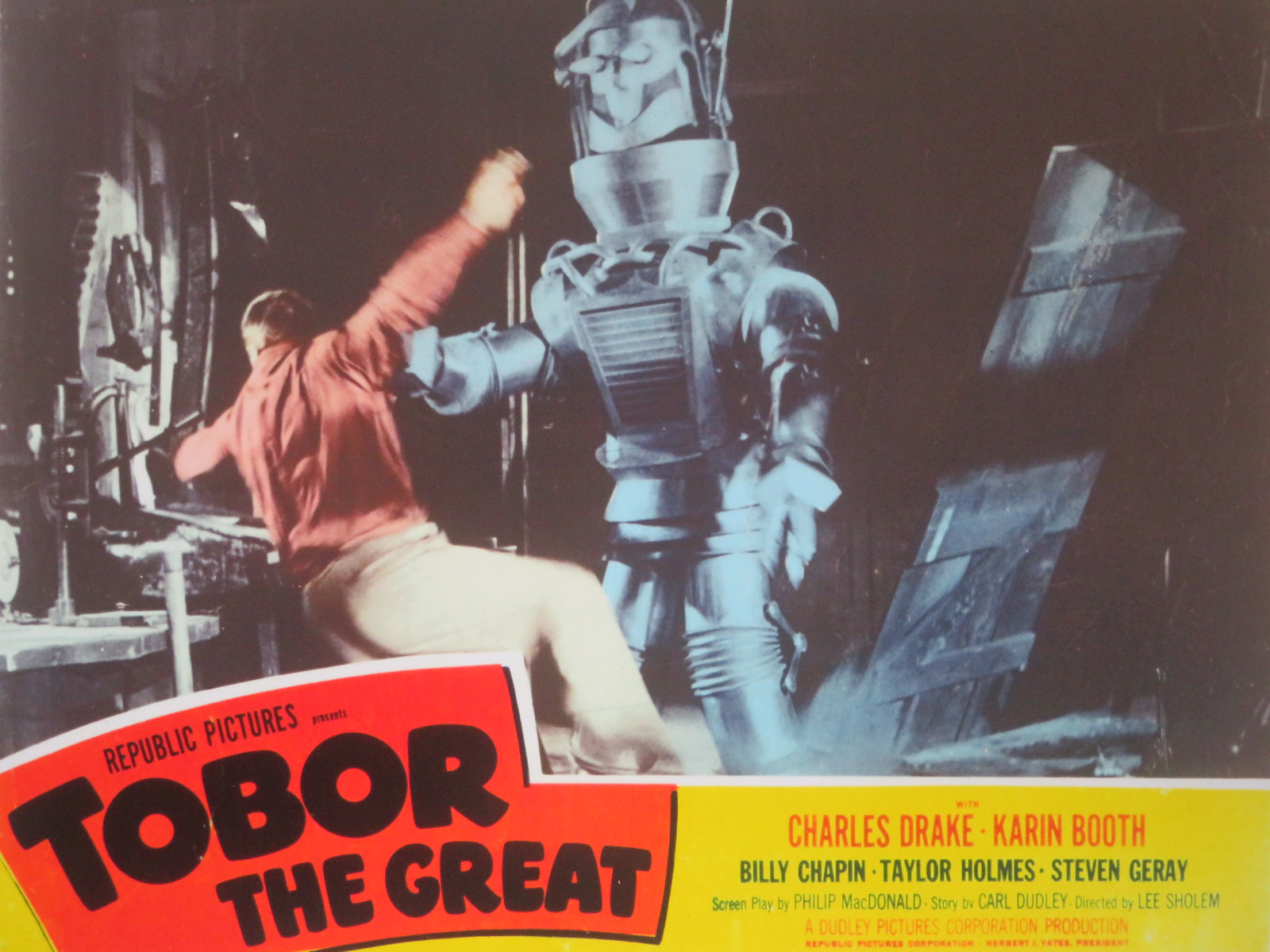The poster image is an old-fashioned movie poster from Republic Pictures for the film "Tobor the Great." At the top of the poster, there is a still from the movie depicting a light blue humanoid robot standing and knocking down a man who is wearing a long-sleeve red shirt and cream-colored pants, set in what appears to be a dark, eerie environment, possibly a factory or a lab. Below this image, against a red background with black letters, it reads "Republic Pictures presents Tobor the Great." On the right side, names of the cast members—Charles Drake, Karen Booth, Billy Chapin, Taylor Holmes, and Stephen Gere—are listed against a yellow background. Additional credits include a screenplay by Philip MacDonald, with a story by Carl Dudley and direction by Lee Sholem. In smaller text at the bottom, it mentions Dudley Pictures Corporation Productions.